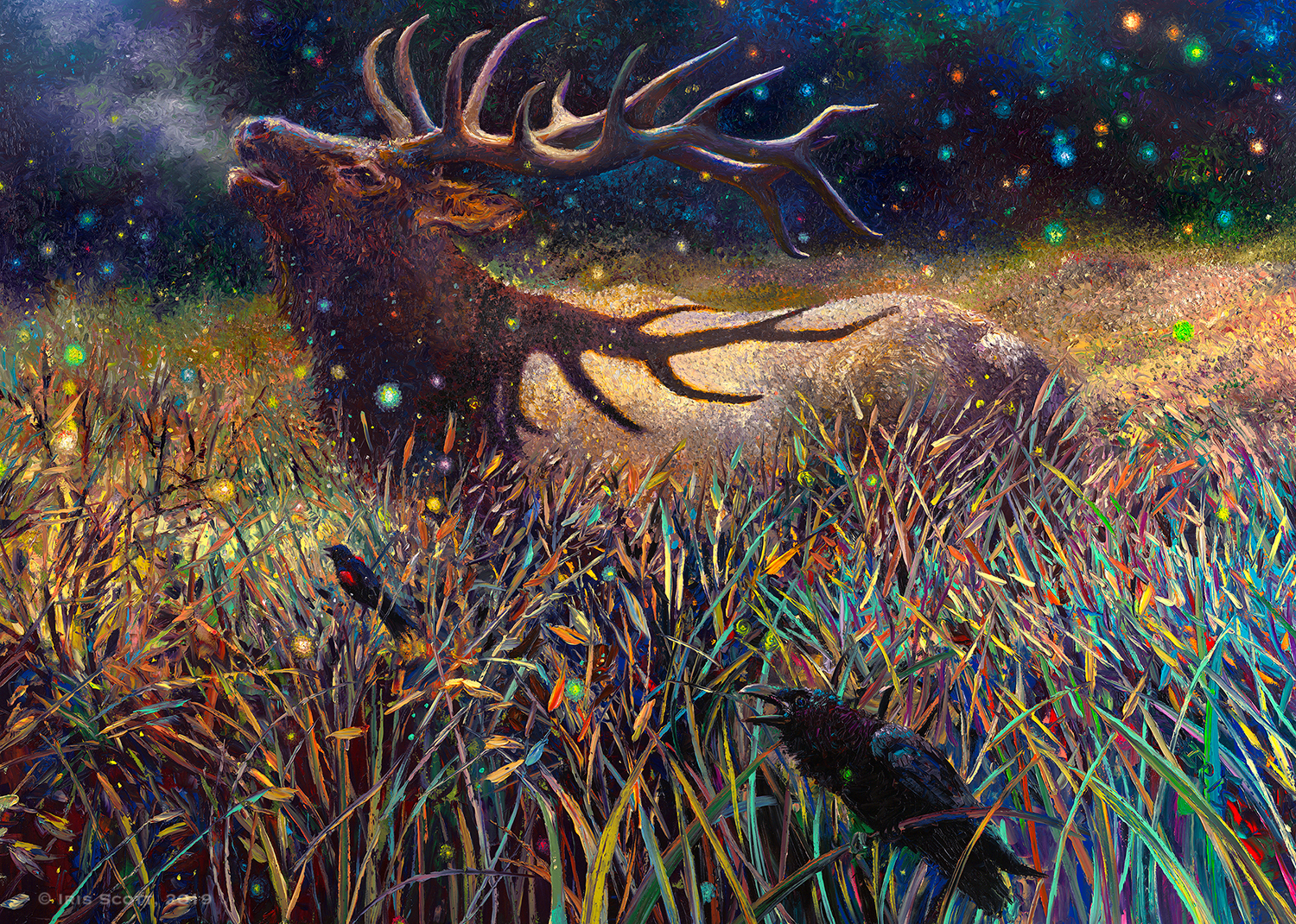This painting, possibly a digitally created graphic design, captures a majestic nighttime scene under dark, star-studded skies. Dominating the center is a grand stag with impressive antlers, standing regally in a shimmering, colorful field. The stag's head is lifted towards the vibrant cosmic sky, its partially open mouth exhaling visible breath. Surrounding the stag, fireflies of various hues—green, blue, orange, red, yellow, and gold—illuminate the scene with their ethereal glow. Below, the field is alive with iridescent weeds and grasses that add to the enchanting atmosphere. Two black ravens, one prominently placed near the viewer, stand among the vibrant flora, both seemingly engaged in cawing. The intricate details and lush colors of the painting blend to create a mesmerizing representation of nature's nighttime chorus.